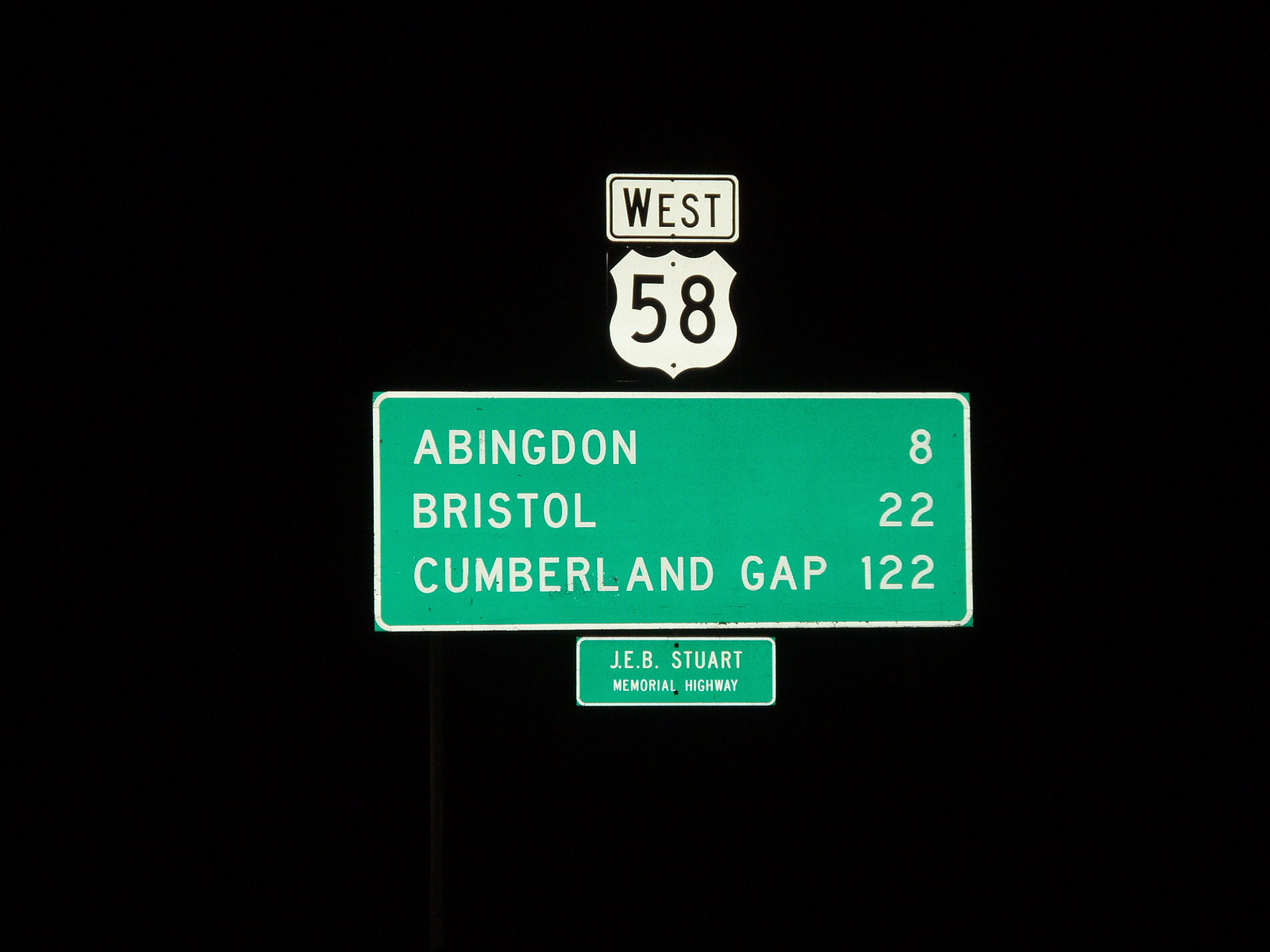This night-time highway image was likely captured from the road with a jet-black background, making only the signs visible. Dominating the center of the image, a series of road signs are illuminated. At the top is a rectangular white sign outlined with a thin black line, featuring the word "West" in bold black letters. Directly below it, a white shield symbol displays the numbers "58" in black, designating Highway 58. Following this, a large green rectangular sign with a thin white border clearly indicates distances to various towns in all-capital white letters: "Abingdon 8," "Bristol 22," and "Cumberland Gap 122." Lastly, a smaller green rectangular sign beneath it, outlined in white, reads "J.E.B. Stewart Memorial Highway" in all-capital white letters. The absence of any visible poles or vehicles, combined with the pitch-black background, intricately isolates these signs, focusing attention purely on their directional and memorial information.